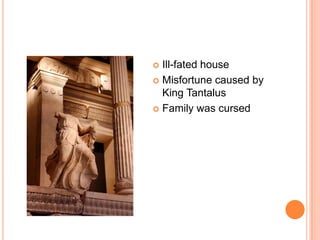The image on the PowerPoint slide appears to be a nighttime photograph of an ancient statue, potentially made of marble, situated in front of a sizable building with tall pillars and lights atop. The statue, headless and missing a left foot and right arm, is draped in a large robe covering most of its figure. The background includes what seems to be a family crypt with a brown door. To the right of the statue, there are several bullet points labeled "Ill-Fated House," "Misfortune Caused by King Tantalus," and "Family Was Cursed," indicating these may be explanations provided during an oral report. The slide features a white background with orange borders and a small orange circle at the bottom right corner.